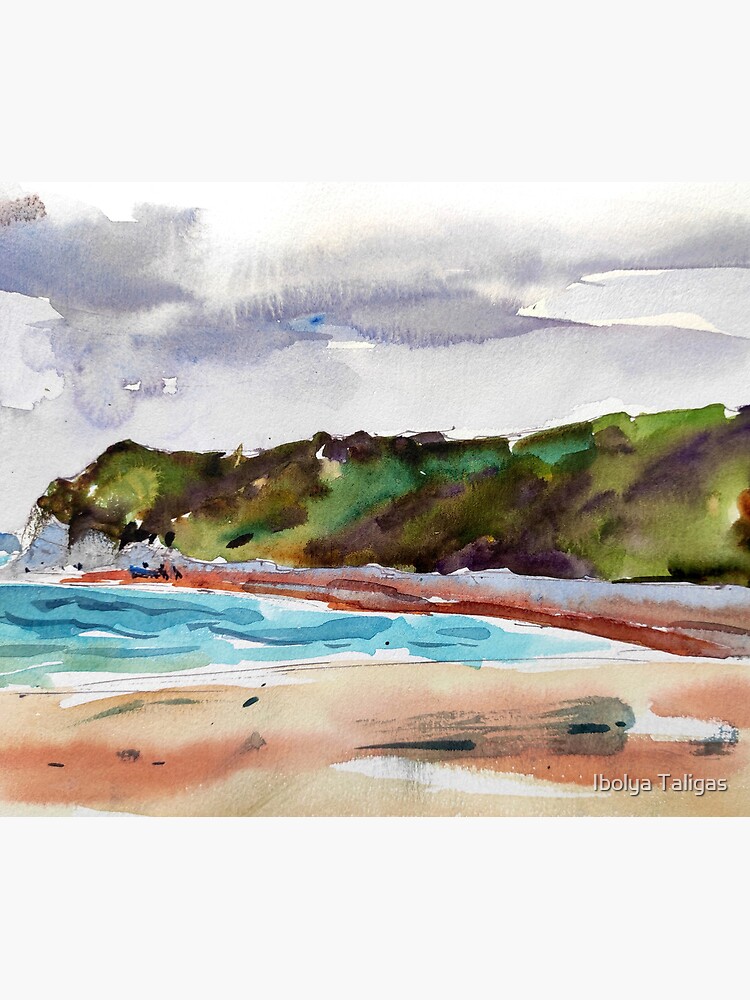This watercolor painting, created by Ibolya Taligas, depicts a beach scene with a detailed and vibrant landscape. The foreground showcases a sandy shore with hues of light brown, beige, and deep red. The turquoise blue water stretches out, reflecting different shades of blue. In the background, a green grassy hill or mountain range emerges, painted with various greens and hints of brown, suggesting a lush environment. The sky above is a mix of dark gray clouds and lighter shades of purple and white, indicating an impending storm. The use of watercolor, possibly mixed with pencil, creates a less realistic, but beautifully smudged and expressive portrayal of a stormy daytime beach scene.